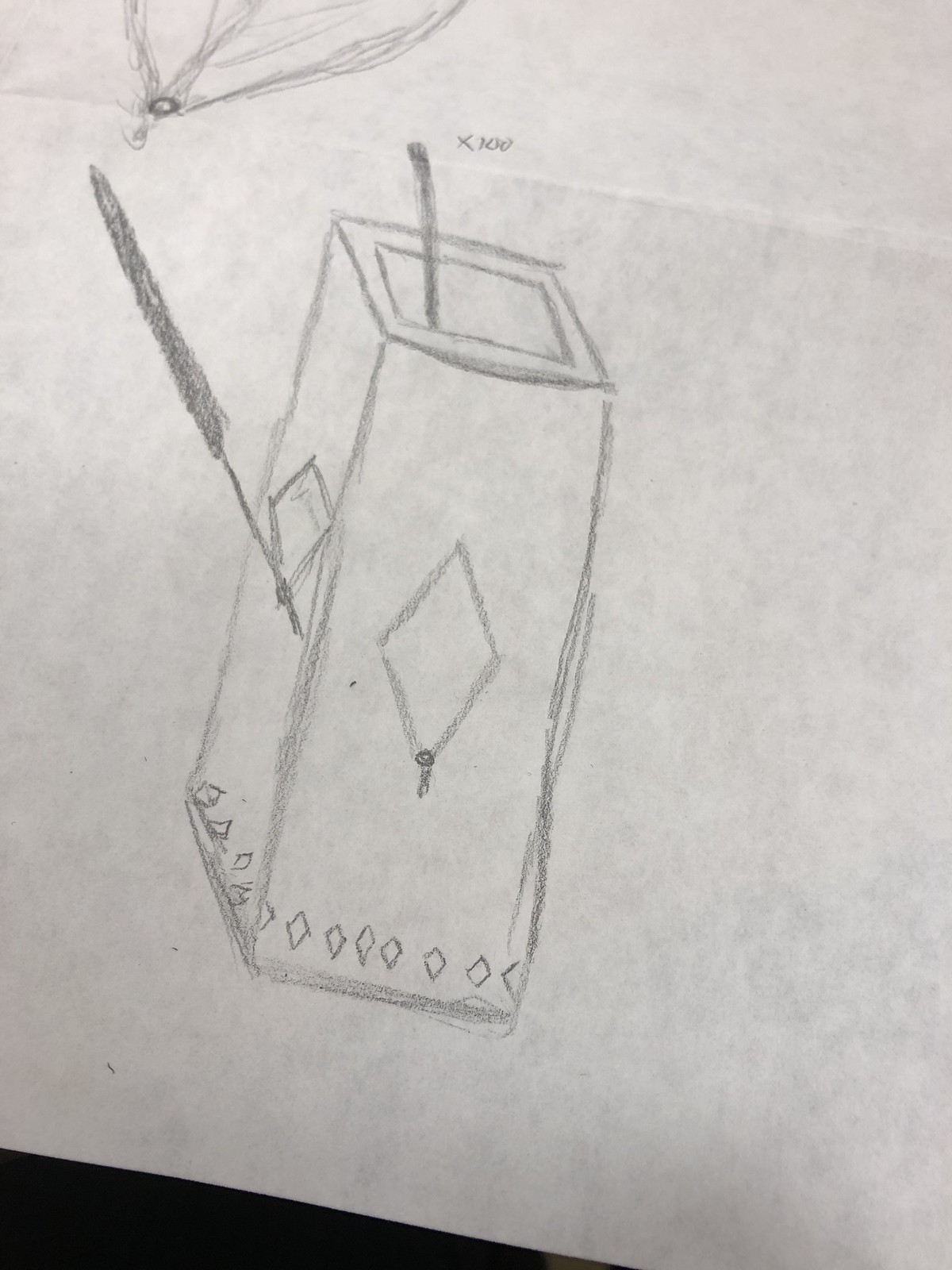A meticulously detailed pencil drawing is showcased, executed on either white or gray paper. The composition features a rectangular structure with a prominent diamond shape at its core, radiating angular extensions. The intricate design evokes the image of a lantern, adorned with diamond patterns centrally and at the base. The drawing employs perspective techniques to give it a three-dimensional, cubical appearance, adding depth and complexity to the otherwise flat rectangular shape.